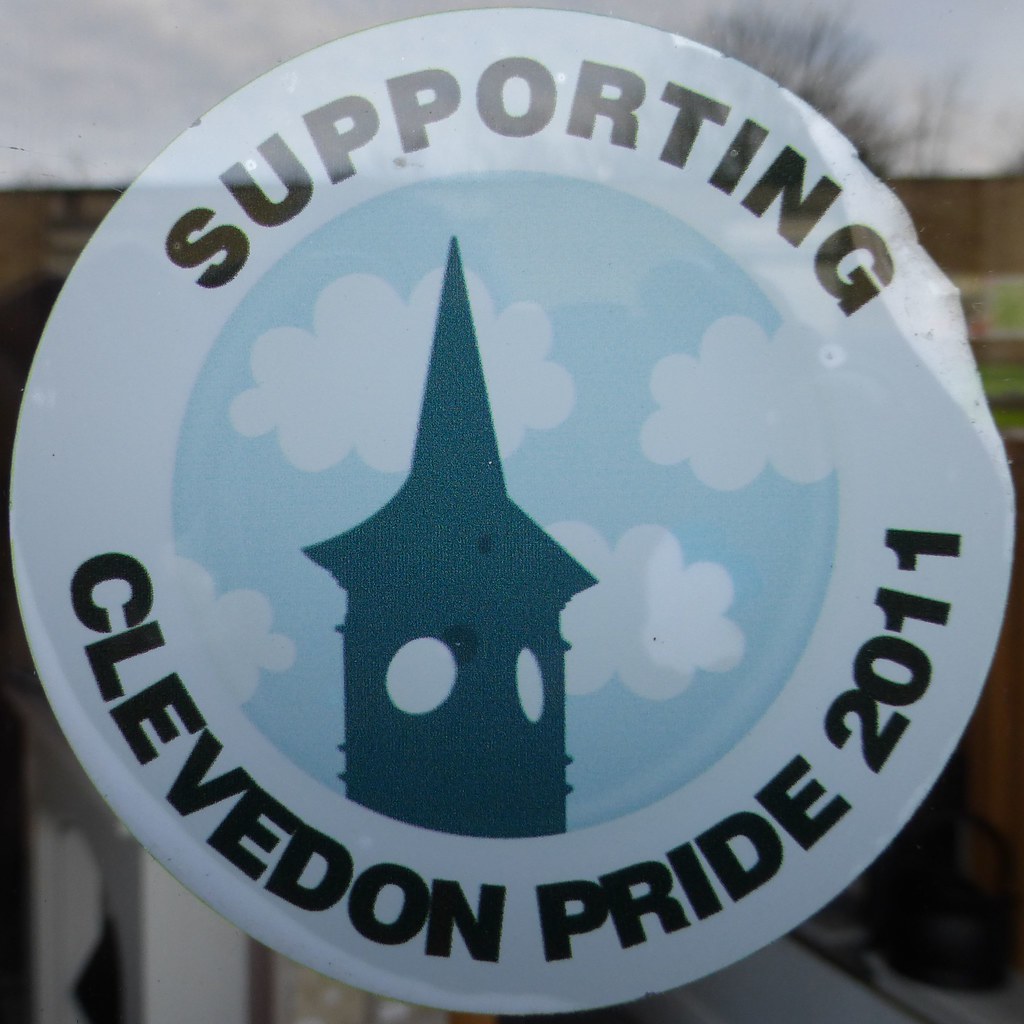The image captures a close-up photograph of a white circular sticker affixed to a glass window. The sticker features the word "SUPPORTING" in black capital letters along the upper arc and "CLEVEDON PRIDE 2011" in black letters along the lower arc. The center of the sticker showcases a light blue circle depicting white clouds and a dark blue building that resembles a steeple or a watchtower. The photograph is slightly blurry, and the background appears to be a reflection on the window, showing glimpses of the sky, tree tops, and possibly a brown building with some grass. Additionally, the sticker seems to be peeling off slightly from the window.